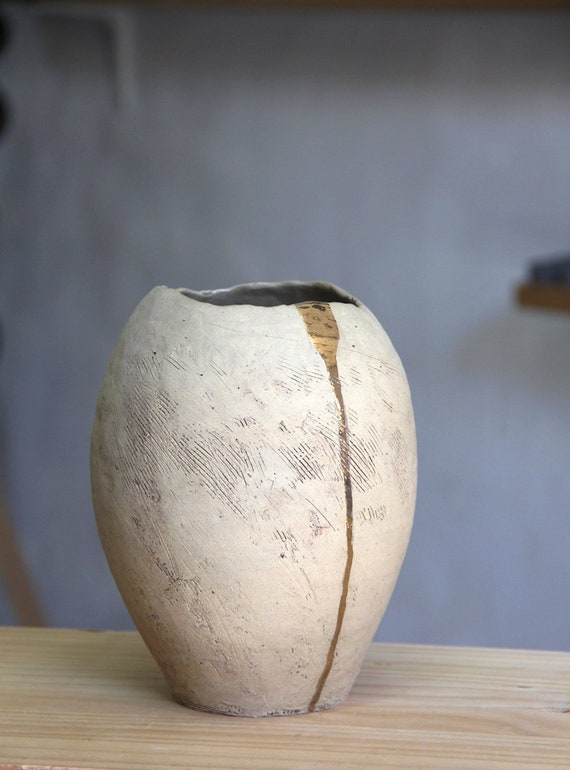The photograph showcases a handmade, rustic clay vase positioned slightly off-center on a light, blonde wooden table with visible wood grain. The background features a warm colonial blue wall, blurred for a shallow depth of field that emphasizes the vase. This oval-shaped vase is predominantly ivory with informal etching revealing a darker color beneath. A striking, narrow gold stripe runs from the un-uniformed opening down the front, becoming more refined as it moves downward, appearing as if the liquid paint naturally flowed to the bottom. The minimalistic composition of the image, with its clean, sparse setting, accentuates the artistry and craftsmanship of the vase.